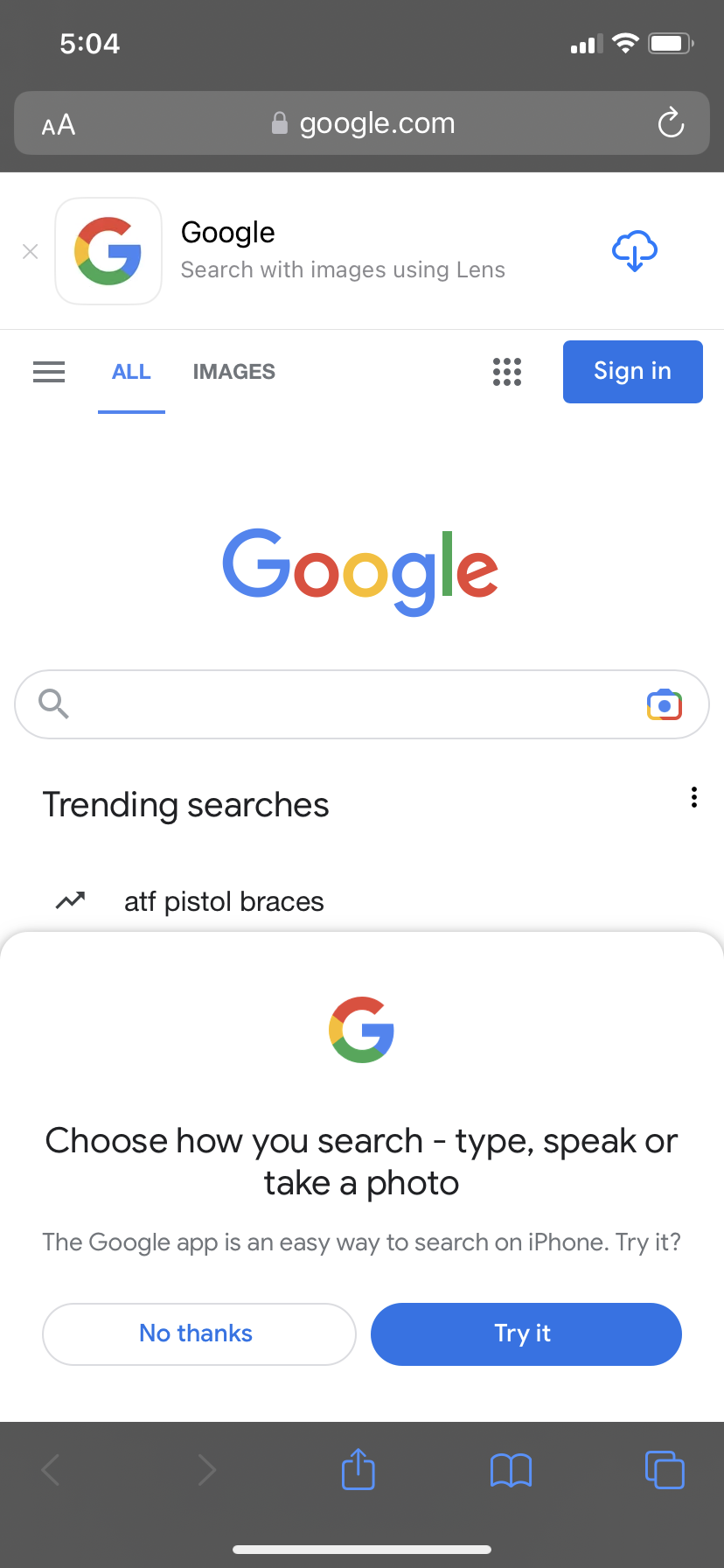The image is a screen capture from a mobile device, showcasing a Google search engine interface. The screen is framed by two horizontal grey bars at the top and bottom. Just beneath the upper grey bar, the iconic Google logo is displayed, featuring a colorful "G" on the left side, followed by the text "Google Search" and the option to search using "Lens" on the right. Adjacent to this, a blue "Sign in" button is prominently visible.

Below this upper section, the main Google logo is central and eye-catching, depicted in its traditional colors of blue, red, yellow, and green. Directly underneath the logo lies the familiar search bar, bordered in a subtle grey outline with a search icon on its left.

Further down the interface, the words "Trending searches" are indicated, suggesting popular or recent search trends. At the very bottom of the page and just above the lower grey bar, there are two interactive buttons. The left button reads "No thanks," while the right button, in a blue oval shape with white text, prompts users to "Try it."